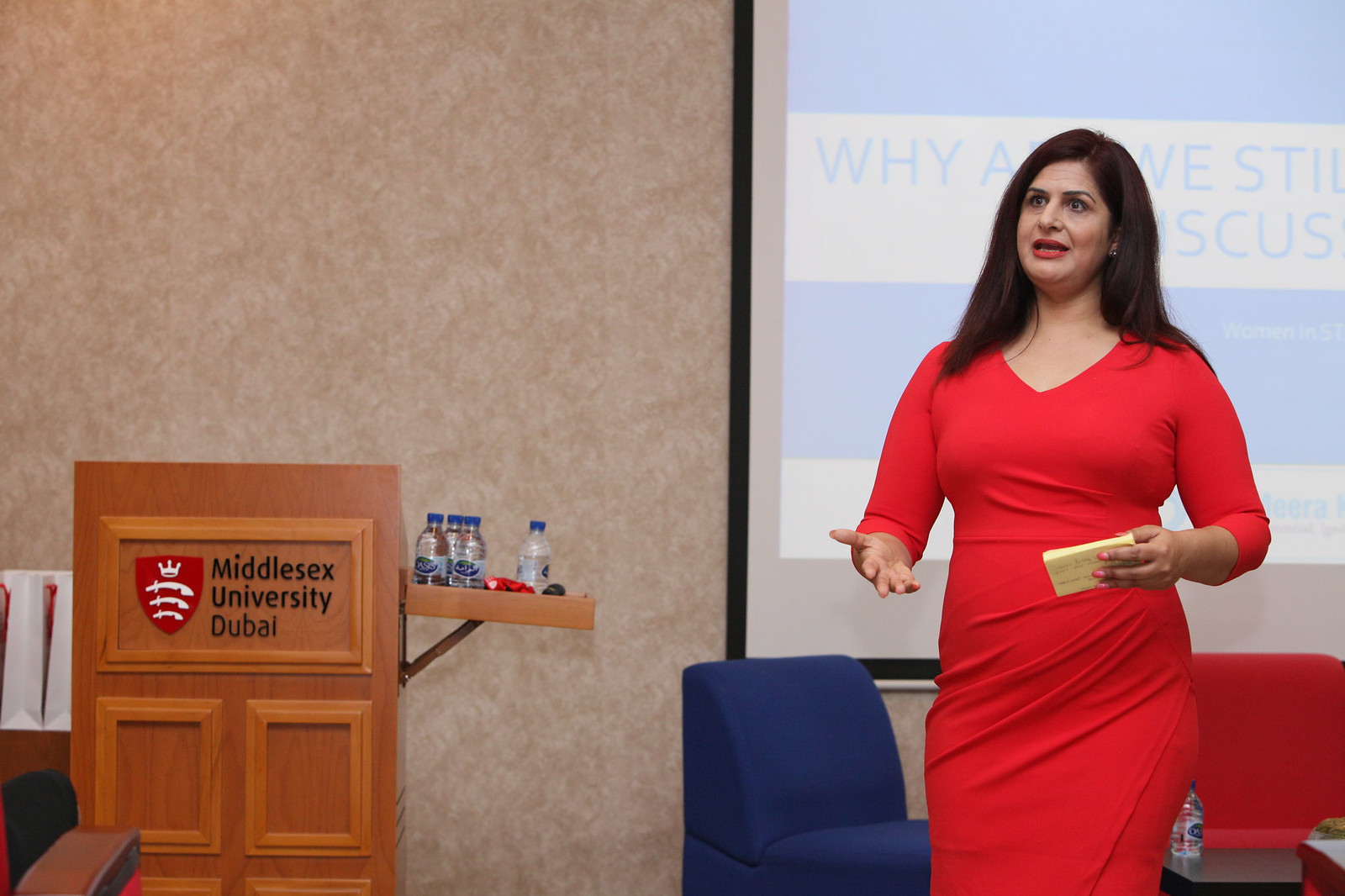In this image, a woman with medium skin tone and long black hair, dressed in a form-fitting, long-sleeved red dress, stands on the right, appearing to give a presentation. She is holding note cards in her left hand while her right hand is raised, palm up at a 90-degree angle, with a surprised or distressed expression on her face. She has red lipstick on, and her hair cascades slightly past her shoulders. 

To her left is a wooden podium with a red shield logo displaying a white crown and three curved swords, labeled "Middlesex University Dubai" in black text. A small shelf extending from the podium holds several bottles of water. Behind the woman, a projection screen with blue and white stripes and partially obscured text reading "Why" is visible. Additionally, a blue chair, a red chair, and a small table with a bottle of water are positioned behind her, against a light tan wall with a subtle design. The overall scene suggests an academic or professional setting, likely a conference or seminar.